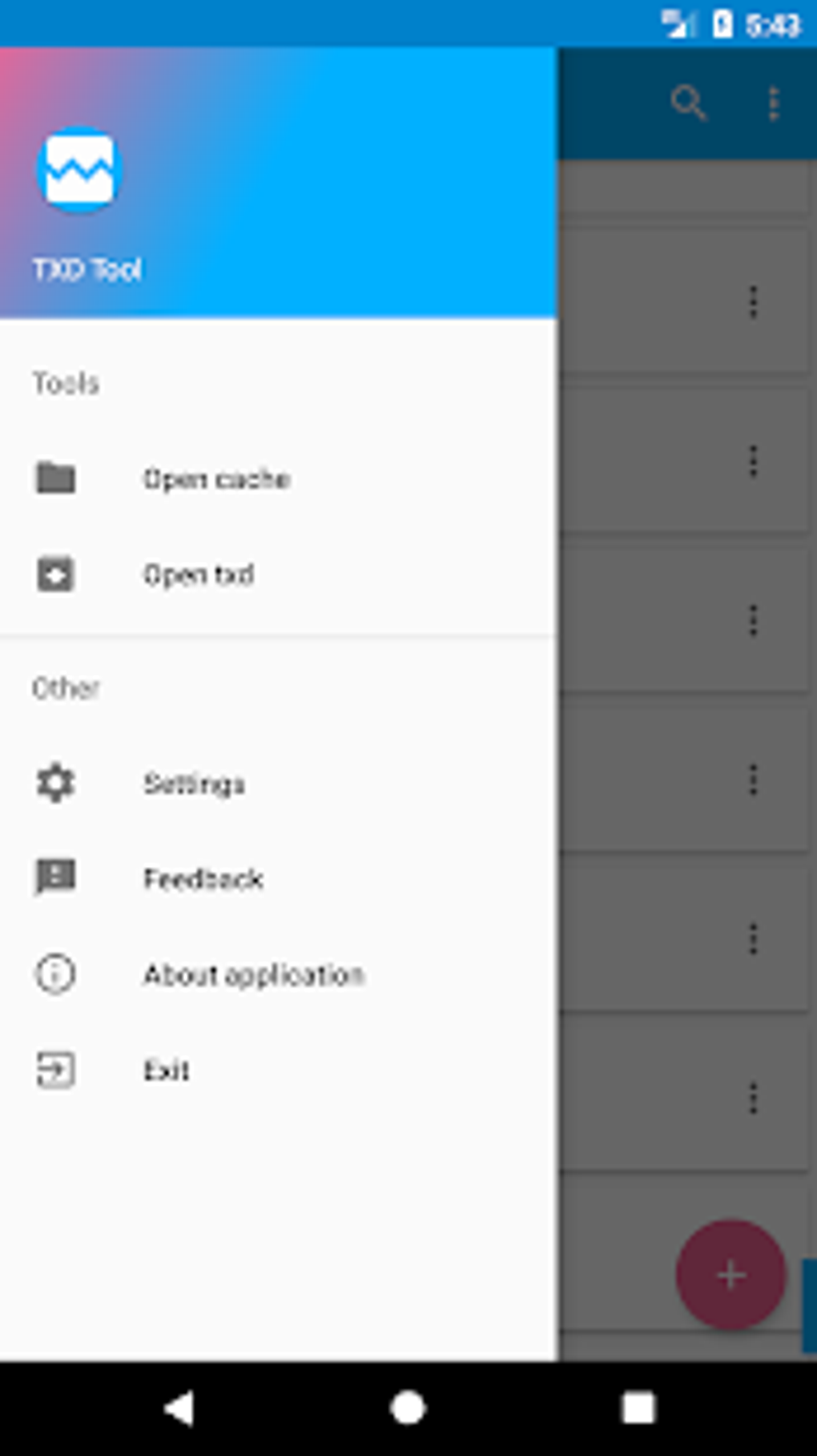In this image, we observe a series of screenshots detailing various aspects of a user interface. The top section of the screen displays the current time, 5:43, alongside a battery icon indicating that the device is charging. The network signal bar is also visible, suggesting connectivity status. On the left side of the screen, there is a menu with several options: "Open Cache," "Open Text," "Settings," "Feedback," "About Application," and "Exit." Beneath this menu, we see the navigation keys and a navigation bar, which guide the user through different sections of the interface. The overall layout provides a comprehensive look at the application's functionality and available user options.